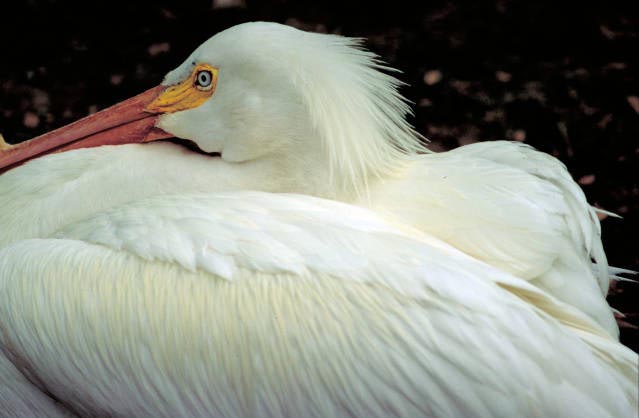This is an up-close photograph of a large white bird, possibly an egret, stork, or pelican. The bird's feathers are entirely white and it features a long, reddish-orange beak. Around its eye is a yellow spot that extends slightly toward its beak. The bird's neck is elegantly curved back, forming a reverse S shape, with its beak appearing to rest on its neck. It is in a seated position with its wings tucked in by its sides. The photograph shows only one eye, as the bird is viewed from the side. The background is a dark, indeterminate color, likely brown or black, and is blurred, making it difficult to identify specific details.